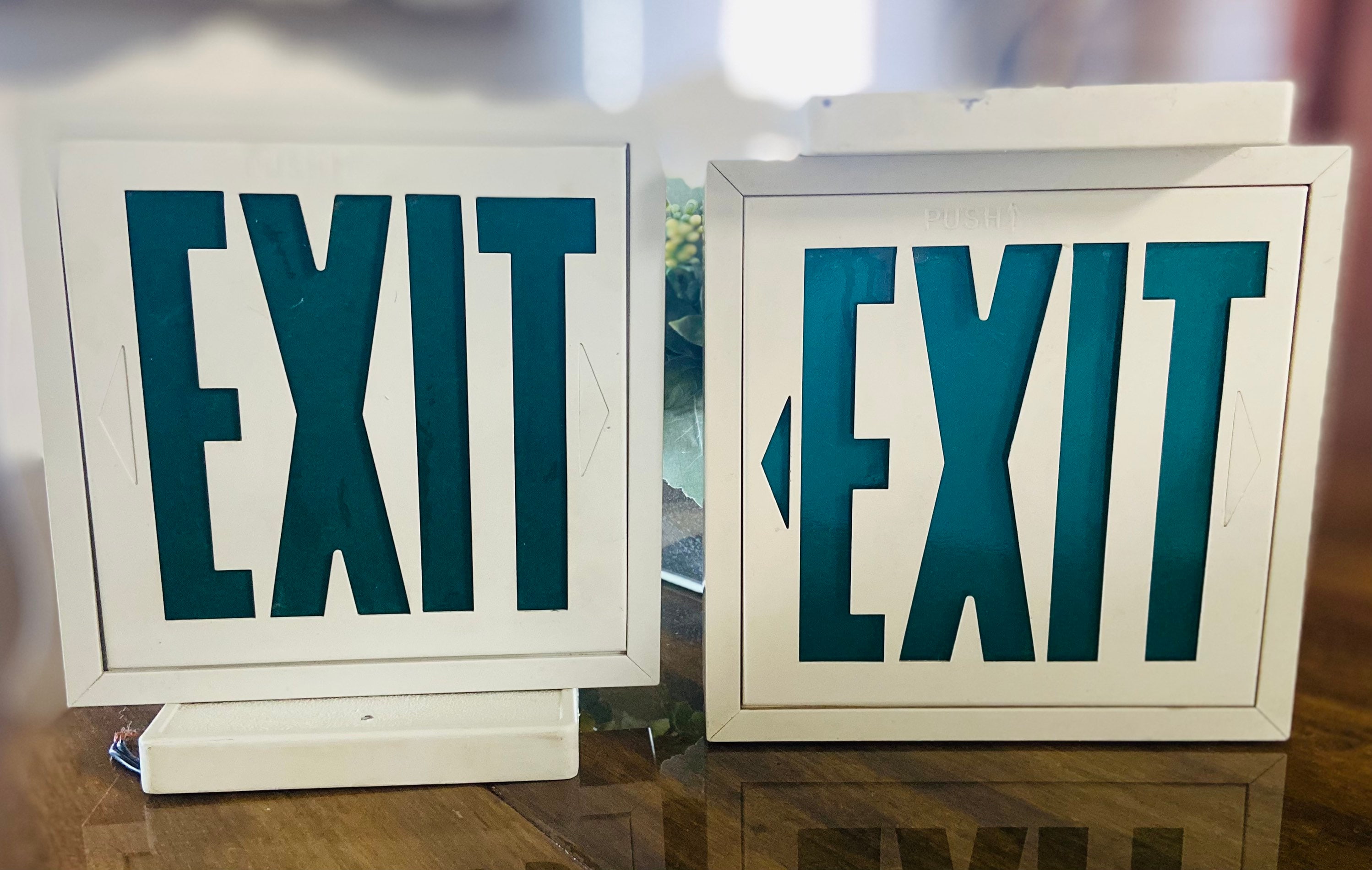This color photograph, taken in landscape mode, showcases two exit signs placed side by side on a glossy wooden table, which reflects the sign on the right. Both signs are encased in white housings, featuring bold text. The left exit sign has dark green lettering without an arrow, and it's designed to be mounted from the bottom. In contrast, the right sign has slightly lighter green text with an arrow to the left and includes a faint "push" marking at the top, indicating its ceiling mount design. An out-of-focus background reveals a hint of yellow flowers.